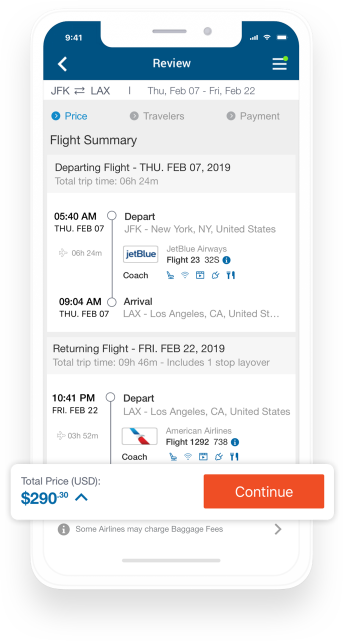In the image, you see the front of a smartphone displaying a blue header at the top. The screen shows the time as 9:41, with a full battery and full Wi-Fi signal bars. Below the header, the word "Review" is prominently displayed. Beneath that are flight details: "JFK ➔ LAX, Thursday, February 7th to Friday, February 22nd."

Following this, there are categories labeled "Price," "Travelers," and "Payment." A section titled "Flight Summary" outlines the departing flight, scheduled for Thursday, February 7th, 2019, with a total trip time of 6 hours and 24 minutes. The flight departs at 5:40 AM from JFK, operated by JetBlue in Coach class, and arrives on the same day at LAX Airport in Los Angeles, California.

The returning flight on Friday, February 22nd, 2019, is detailed next. This trip includes one stop and has a total duration of 9 hours and 46 minutes, departing from LAX in Los Angeles, California.

At the bottom of the screen, there's a white bar that highlights the total price on the left, indicated as "Total Price, USD" with an amount of "$290" displayed below it. On the right side of the white bar, there's a long orange button labeled "Continue."